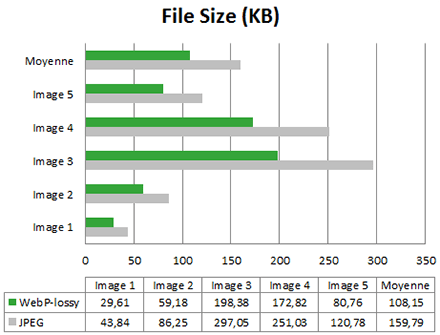This infographic visually compares the file sizes of various images in kilobytes (KB) using two different formats: WebP Lossy and JPEG. At the top, the title "File Size (KB)" is prominently displayed in bold. The horizontal axis (x-axis) at the bottom is labeled with file sizes ranging from 0 to 350 KB in increments of 50 (0, 50, 100, 150, 200, 250, 300, 350). 

The vertical axis (y-axis) represents different images labeled as image 1 through image 5 from bottom to top, though it seems there might be a typo or mislabeling, with "MoYen" at the top. 

Green lines on the chart depict the file sizes for WebP Lossy format, while gray lines represent the JPEG format. Specific file size values are provided for each format and image, as follows:

- Image 1: WebP Lossy - 29 KB; JPEG - 61 KB
- Image 2: WebP Lossy - 59 KB; JPEG - 18 KB
- Image 3: WebP Lossy - 198 KB; JPEG - 38 KB
- Image 4: WebP Lossy - 170 KB; JPEG - 282 KB
- Image 5: WebP Lossy - 80 KB; JPEG - 76 KB

Additional values are included but are not clearly associated with specific images:
- WebP Lossy: 108 KB, 15 KB, 43 KB, 84 KB, 86 KB, 25 KB, 29 KB, 05 KB, 250 KB, 103 KB
- JPEG: 120 KB, 78 KB, 159 KB, 79 KB

These values visually demonstrate how the file sizes differ between WebP Lossy and JPEG formats across multiple images.